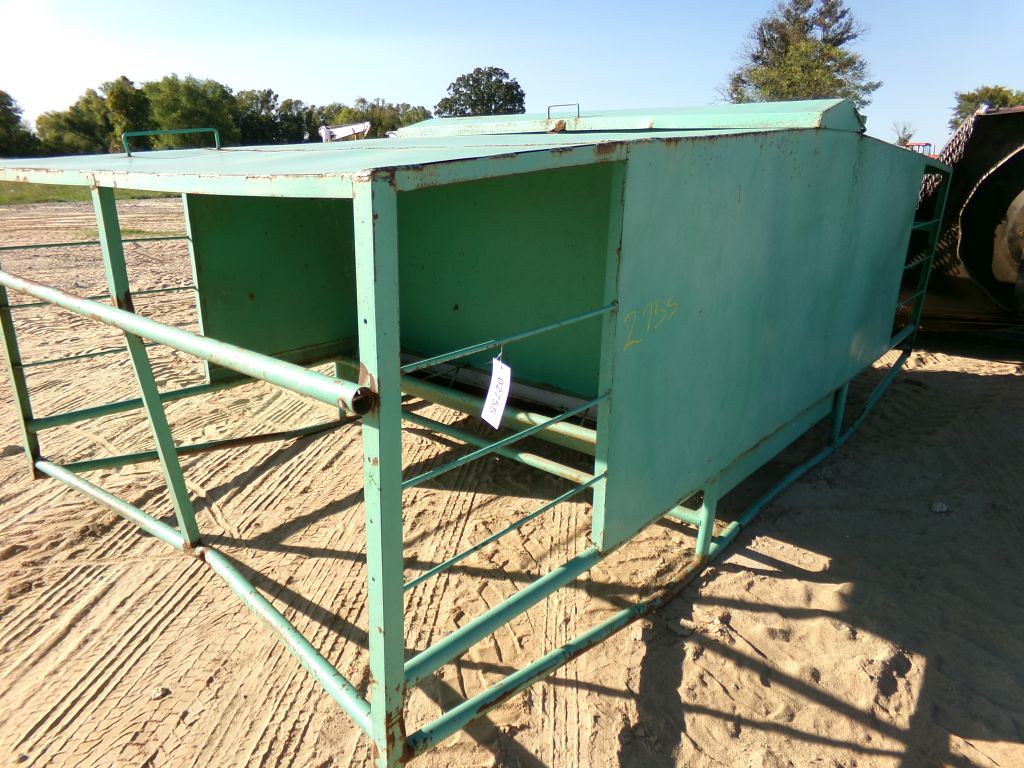The image depicts a dilapidated, mint green metal container building, sitting on a sandy dirt terrain with tire tracks crisscrossing beneath it. This rusted structure, possibly used for farming or as an animal enclosure, features an enclosed rear section and an open front with green metal bars and fencing, some of which appear broken and in need of repair. A tag hangs from one of the bars, marked with the number 2755. The background showcases a line of leafy trees under a clear, powder blue sky, framing the scene and hinting at a rural or farm setting.